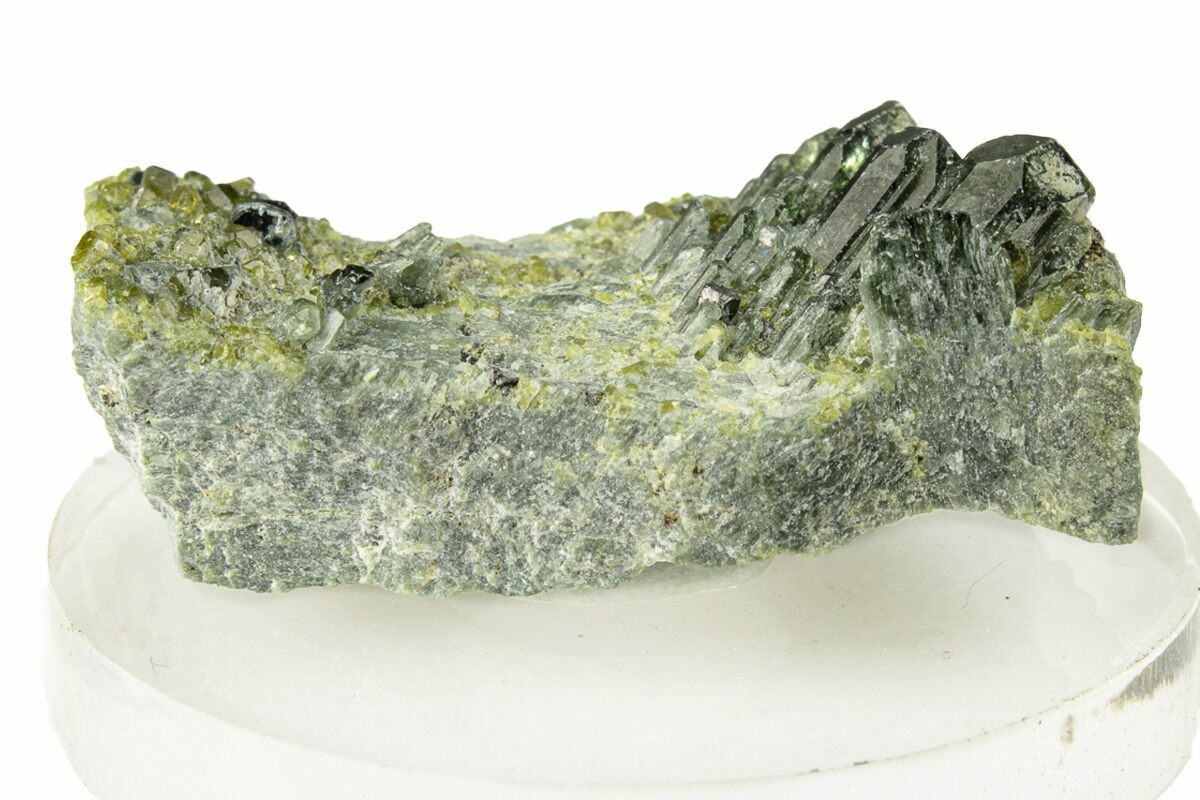This image features a detailed close-up of a geological specimen, possibly a gemstone or crystal, displayed on a transparent circular glass platform. The rock itself exhibits a stunning mix of colors, including various shades of green, yellow, brown, and hints of gray. Its surface is shiny and may suggest it is composed of minerals like turquoise or tourmaline, characterized by intricate cut structures reminiscent of a geode. The specimen is thicker at the ends and lower in the middle, indicating a natural formation or a specific section cut out for display purposes. The photograph appears to have been taken indoors in a controlled setting, potentially for a museum, lab, or website showcasing minerals. The background is plain white, with no additional items or text, highlighting the rock's unique and beautiful features on its clear glass base.